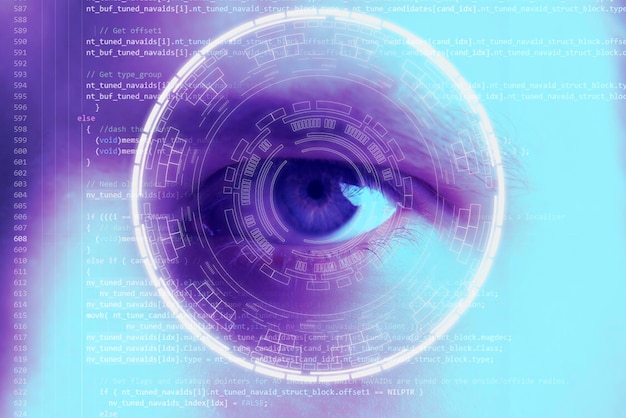The image is a horizontally oriented rectangle. Dominating the center is a circle featuring a detailed, bluish-purple eye with a black pupil at its very core. This eye is rendered with meticulous attention to elements like the eyebrow, eyelids, and eyelashes, giving it a realistic appearance. Overlaying the circular section is an intricate pattern of white boxes arranged in concentric circles, creating a striking visual frame around the eye.

Layered atop this central design is a stream of programming code, running horizontally from left to right. On the far left edge, a line count is displayed, vertically numbering the lines of code starting approximately at 587 and ending somewhere near 623 or 624, though the exact bottom number is unclear. The combination of anatomical detail and digital elements creates a captivating and multidimensional composition, blending the organic with the technological.